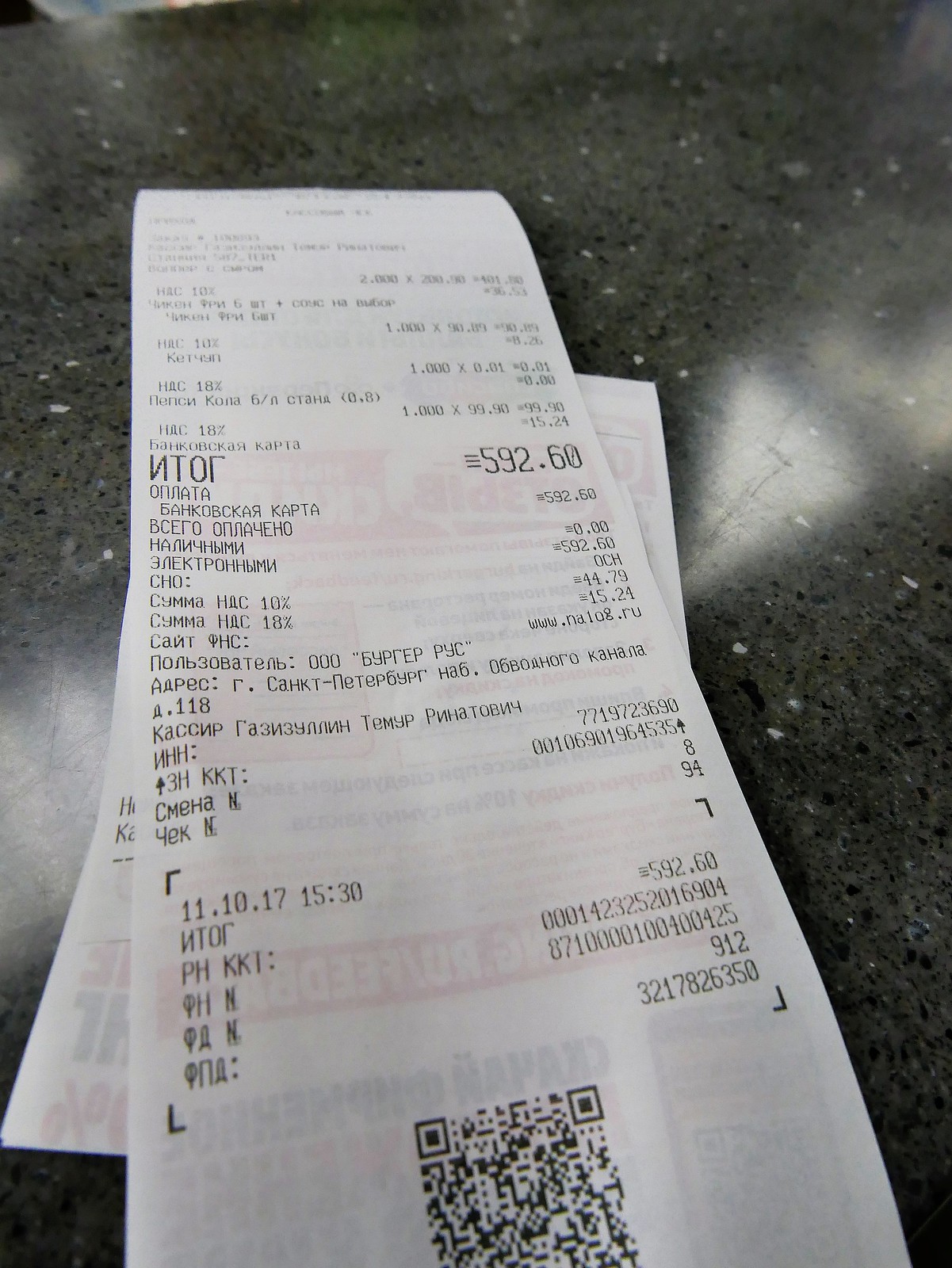A high-resolution, color photograph showcases two receipts, one atop the other, on a reflective, dark gray surface with a marble-like texture featuring black and white specks. The foreground and background of the image are slightly blurred, drawing focus to the center of the top receipt. The prominent receipt, in fair condition and pure white, features black text in the Cyrillic alphabet, suggesting it could be either Greek or Russian. Notable details include the item price of 592.60 in an unspecified currency and a QR code at the bottom for additional information. The secondary receipt underneath is mostly obscured, with only a few letters visible.